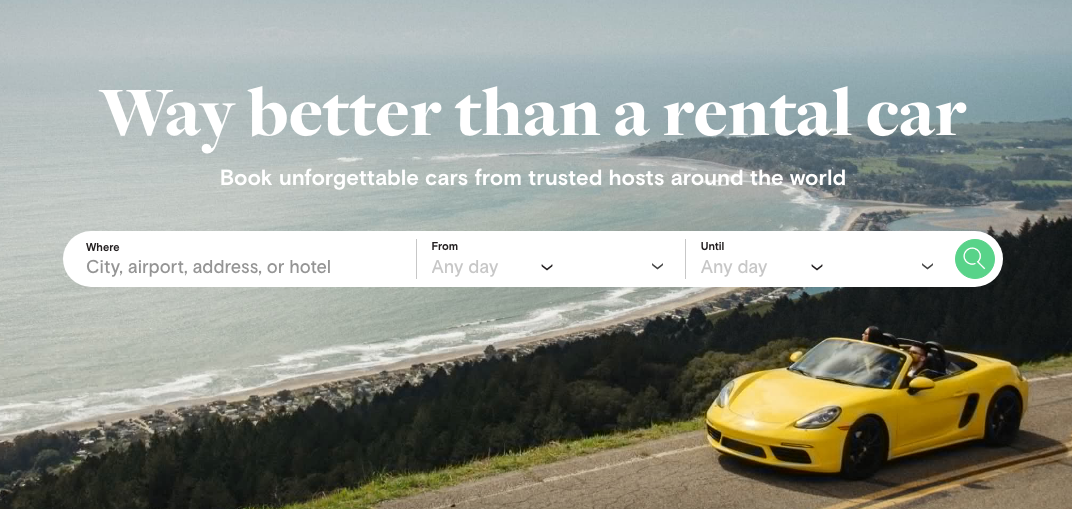This is a left-to-right horizontal image depicting an advertisement for a car rental service, ideal for viewing on a smartphone or computer. The serene background features a seamless blend of sky and water in shades of grayish-blue, with a thin strip of trees and a small tan beach area visible near the horizon, creating a tranquil backdrop. Positioned prominently on a road in the foreground is a vibrant yellow convertible occupied by two people in the front seat, enjoying their drive.

Overlaying this scenic view, bold white text declares, "Way better than a rental car." Beneath this in slightly smaller, less bold white text, the slogan reads, "Book unforgettable cars from trusted hosts around the world." Below the text, there is an interactive search bar with the options for "City, airport, address, or hotel" and fields labeled "From" and "Until" where users can select their preferred dates from dropdown menus. Completing the interface is a green search button featuring a magnifying glass icon, inviting potential customers to begin their search.